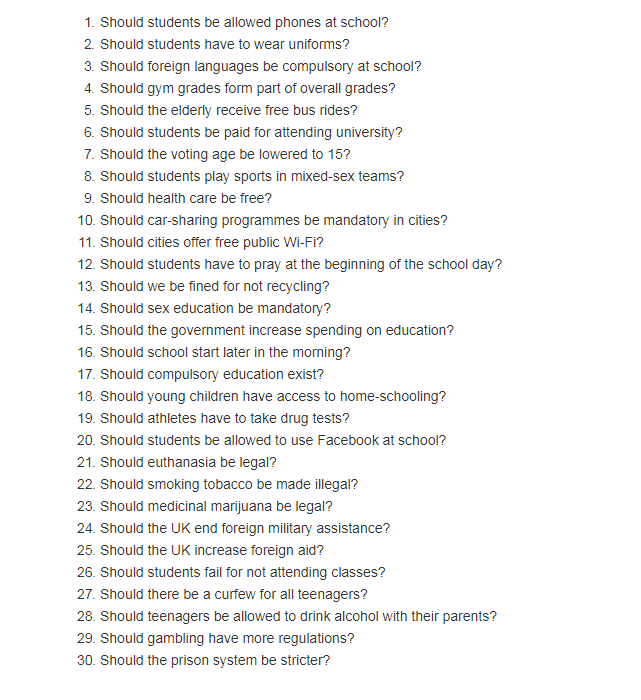A cropped image displays a list of 30 questions arranged vertically, numbered from 1 to 30. The questions are written in very small black font, with each number followed by a period and a space, preceding the actual question. There are no answers provided, nor any dropdown boxes or guides accompanying the questions, making the document appear as a straightforward printout sheet. The questions seem to cover a range of diverse topics, akin to those one might ask in a search engine. For instance, question number 1 is "Should students be allowed...," questions concerning societal issues like "Should healthcare be free?" and environmental concerns such as "Should we be fined for not recycling?" appear on the list. Question number 26 specifically asks, "Should students fail for not attending classes?" The assortment of questions indicates a random yet thought-provoking compilation likely intended to spark discussion or serve as prompts for further inquiry.